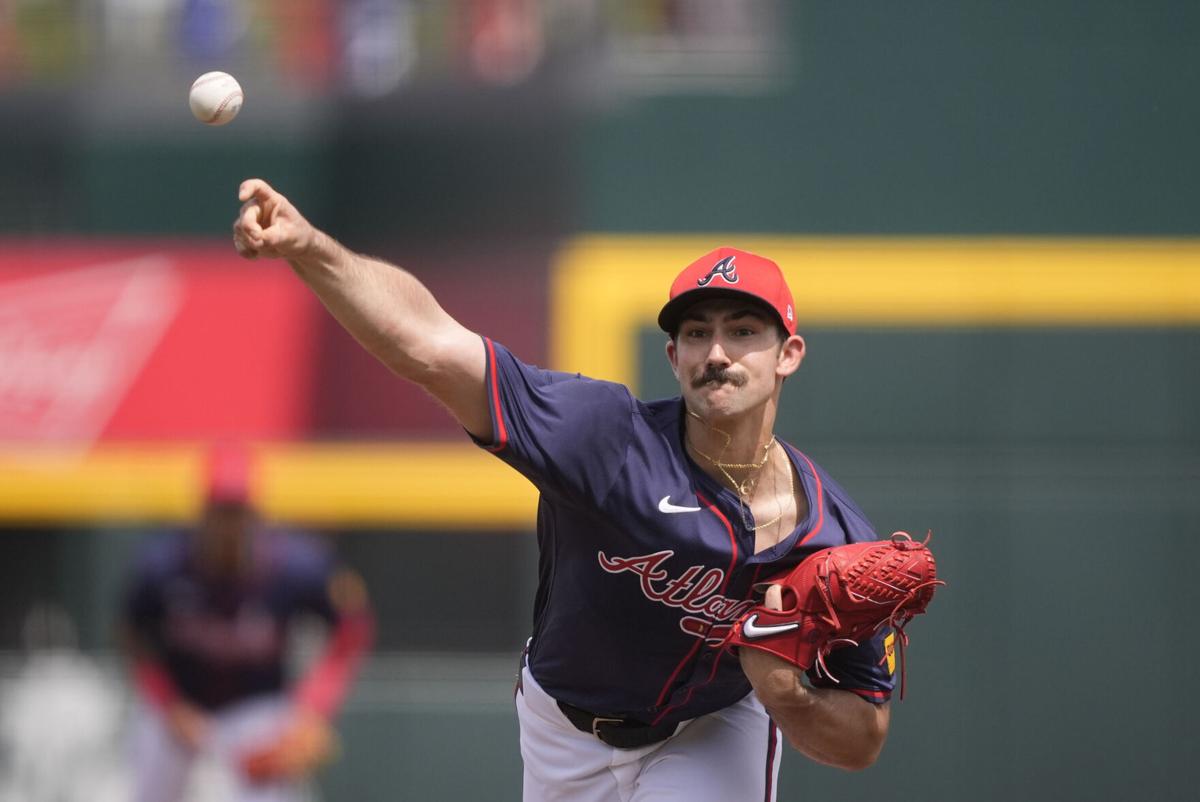This detailed color photograph captures a dynamic action shot of an Atlanta Braves pitcher mid-throw on the mound. The pitcher, who appears to be around 35 years old with a brown mustache, is adorned in a dark blue Atlanta Braves jersey trimmed with red, featuring "Atlanta Braves" on the front and a white Nike swoosh in the upper right corner. He wears white baseball pants with red stripes, secured by a black belt. The player's red cap, emblazoned with the iconic Atlanta Braves "A" logo, contrasts sharply with his dark blue uniform. The image also highlights the red baseball glove on his left hand, which bears a Nike swoosh, while his right hand is captured in the precise moment as he releases the ball, his crooked index finger adding to the intensity of the shot. Around his neck, two gold chains glint in the light. The background of the image is beautifully blurred, showing segments of the stadium with a dark aqua wall adorned with yellow and red banners, and another Braves player, likely the catcher, poised attentively, enhancing the focus on the pitcher in this representational realism photograph.